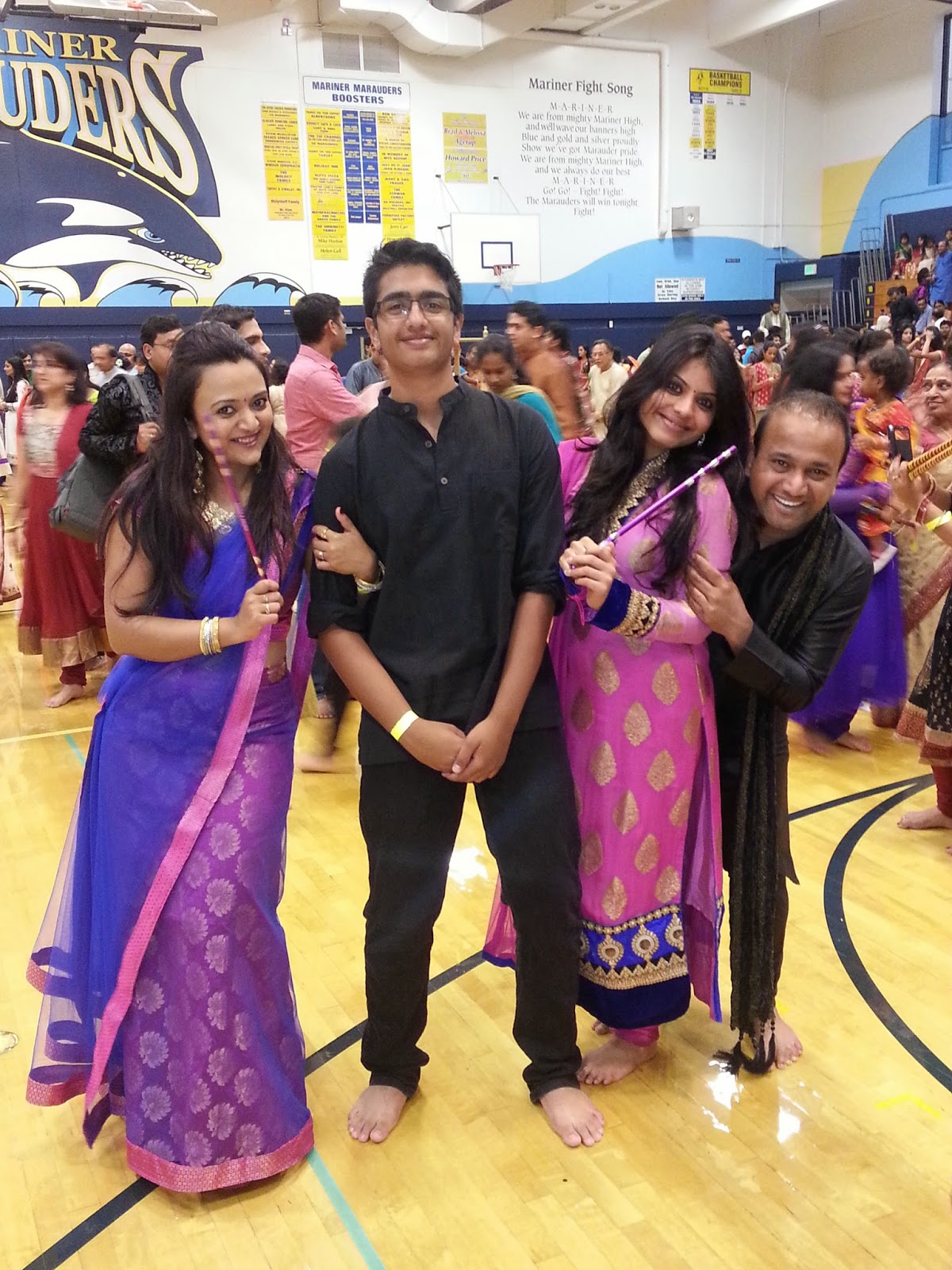The image depicts a bustling scene inside a gymnasium, likely at a high school in either India or America, as suggested by the cultural attire and overall setting. The gym's polished hardwood floor gleams with a glossy finish, scattered with traces of paint, hinting at its use as a basketball court. A large crowd, primarily positioned at the center of the image, consists of well-dressed individuals; men in button-down shirts and women in traditional Indian dresses of vibrant colors like purple, pink, and blue. The diverse palette extends into the background, with additional hues such as light blue, black, red, maroon, yellow, dark blue, brown, and beige visible. Among the group stands a young barefoot Indian individual. The participants are gathered close together, exuding happiness and smiling, lending to a celebratory atmosphere. Although the exact nature of the event is unclear, it might be a graduation, sports victory, or academic achievement, reinforced by the "Mariner Fight Song" poster on the wall. The scene, framed in a vertical rectangular format, encapsulates a moment of communal joy and cultural pride.